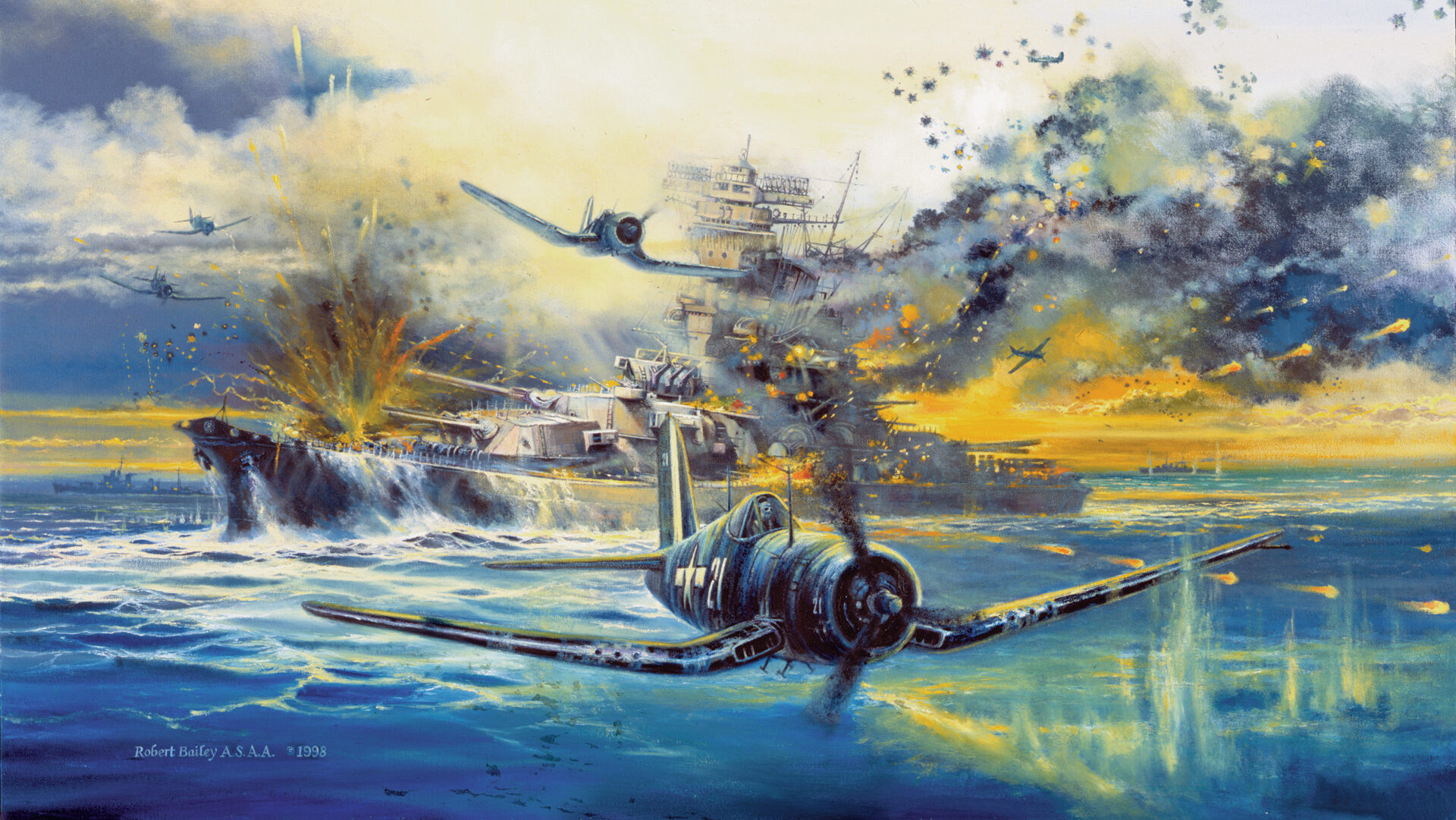This vivid color illustration depicts a dramatic and intense battle at sea, likely inspired by scenes from World War I or World War II. Dominating the background is a massive, modern battleship engulfed in explosions and fire, indicating a direct hit from an aerial attack. Waves splash onto the burning deck while artillery shells explode around the ship. The sky is filled with puffs of smoke and cloud formations, with a total of five black planes engaged in the conflict. In the foreground, a prominently featured airplane, marked with the number "21" and bearing a circular logo with a dark background and white star, swoops down towards the viewer just above the water, seemingly faltering and on the brink of crashing. More ships can be spotted in the background, adding to the chaos of the battle scene. The painting is rendered in shades of blue, gray, and yellow, with vibrant orange flames, giving it a striking and memorable visual impact. The bottom left corner is signed by the artist, Robert Bailey, ASAA, dated 1998.